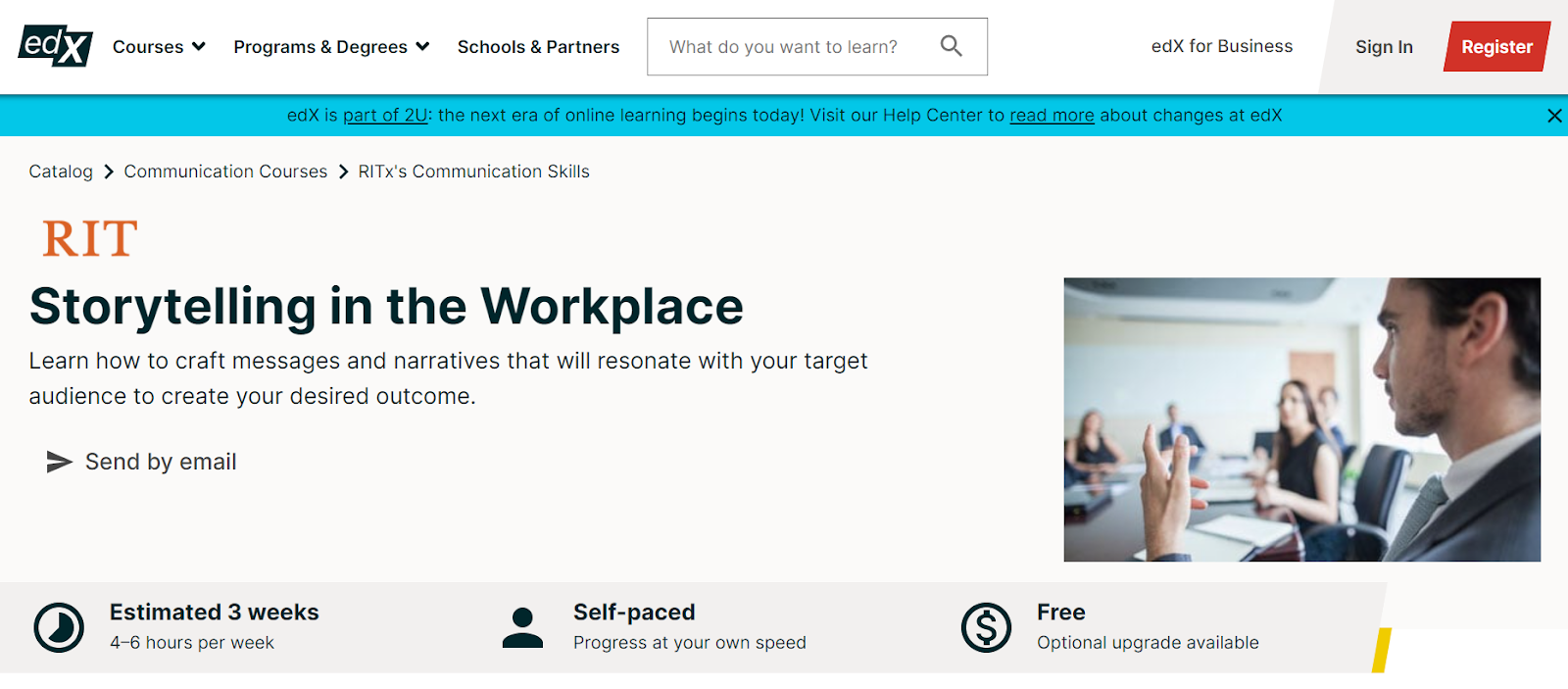The image is a screenshot of the edX website's homepage. On the top left corner, the edX logo is prominently displayed. Adjacent to the logo are navigation links labeled "Courses," "Programs and Degrees," "Schools and Partners," and a search bar with the placeholder text, "What do you want to learn?" On the top right, there are options for "edX for Business," "Sign In," and "Register," with the "Register" button highlighted in white text on a red background. 

Beneath the navigation bar, there's a banner with a blue background stating, "edX is passed off to you. The next era of online learning begins today. Visit our help center to read more about changes at edX."

In the main section, a highlighted course from RIT (Rochester Institute of Technology) is featured. The text details a course titled "Storytelling in the Workplace," which teaches how to craft messages and narratives to resonate with target audiences and create desired outcomes. Beside the course description, there's an option to send the details by email.

At the bottom left of the course listing, there are details that the course is estimated to take three weeks, with a commitment of four to six hours per week. The course is self-paced, allowing progress at the student's own speed, and it is free with an optional upgrade available. These texts are written in black on a light grey background.

Above this course description, to the right, there is an image of people engaged in learning activities, underscoring the educational focus of the website.